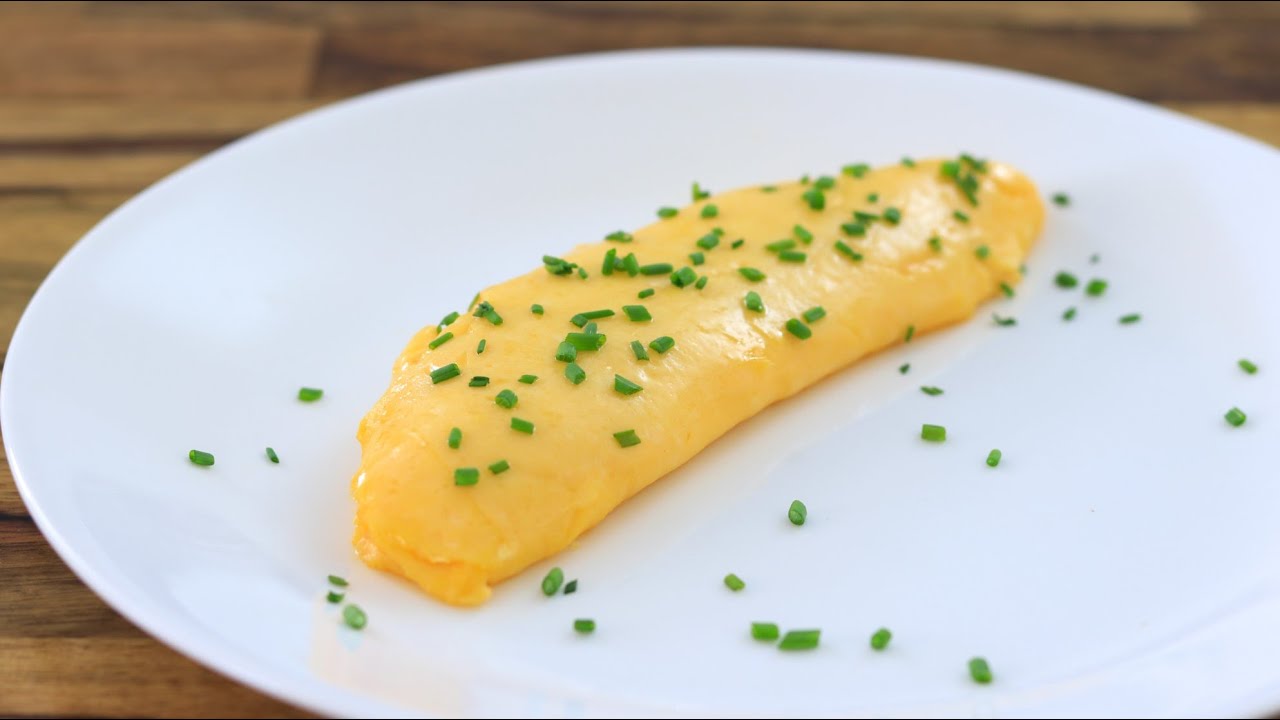The photograph captures a neatly arranged dish of what appears to be a yellow, folded omelette, placed at the center of a white plate. The plate itself rests on a brown wooden surface, which could be a countertop or tabletop. The omelette has a smooth, shiny texture and is shaped like a semicircle. Tiny green pieces, likely chives, are generously sprinkled over the omelette and scattered around the plate. Additionally, there is a slight stain of color visible on the bottom left portion of the plate, adding a touch of contrast to the otherwise pristine white surface.